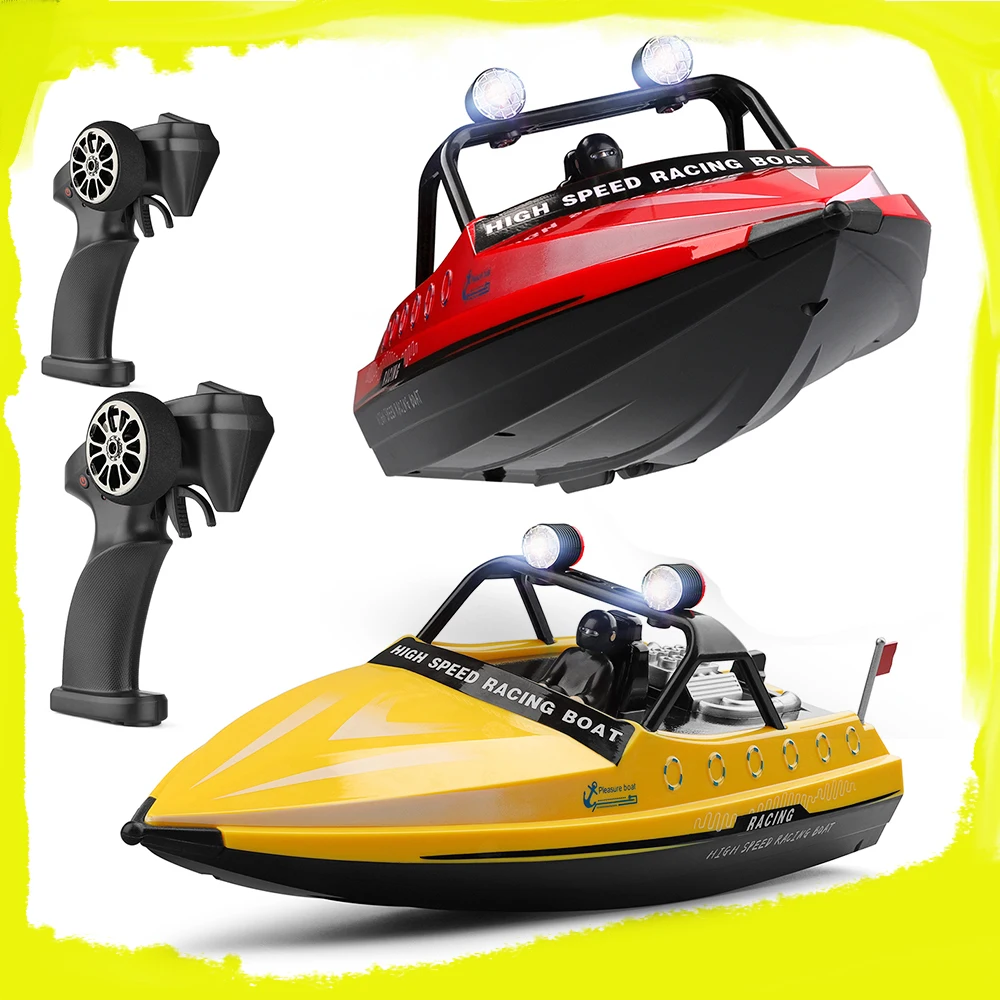The image is a stock photograph featuring two radio-controlled speedboats and their corresponding black remote controls. It is a wide vertical rectangular image with a yellow border painted unevenly around a solid white background. On the upper left corner, there are two black remote controls resembling guns with long handles and wheels on the side, positioning one above the other. 

To the right of the remote controls are two speedboats of identical design but different colors. The upper boat has a red top and a black bottom, with prominent white headlights on a black rectangular pipe across the top, and the words "High Speed Racing Boat" inscribed on its body. Slightly angled upwards, its nose points to the right. The lower boat is similar but features a yellow top and a black bottom, with its nose facing left. Both boats have a small black plastic figurine dressed in a ninja-like full body suit, including a helmet, seated in the driver's position. Additionally, there's a silver flagpole with a red flag on the rear part of each boat.